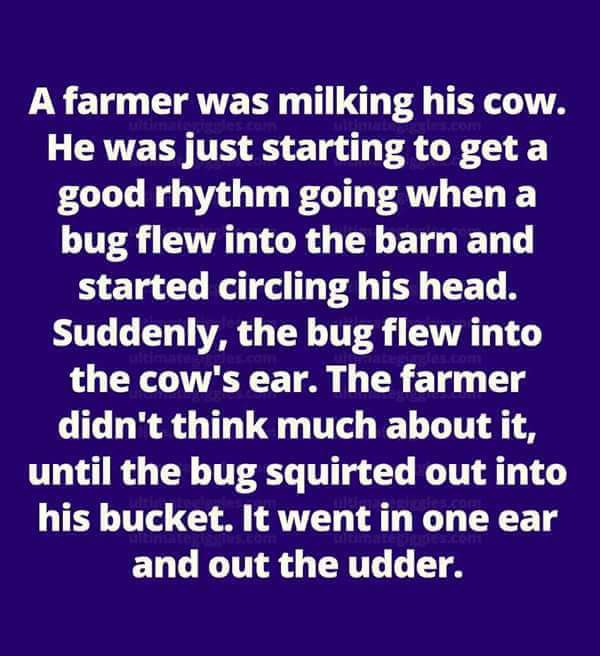In this image, a rectangular background in a dark purplish color showcases white, bold-text centered in the middle. The text narrates a humorous short story: "A farmer was milking his cow. He was just starting to get a good rhythm going when a bug flew into the barn and started circling his head. Suddenly, the bug flew into the cow's ear. The farmer didn't think much about it until the bug squirted out into his bucket. It went in one ear and out the other." The text, appearing somewhat distorted with hints of blurriness between the lines, stands out clearly against the purple backdrop, resembling the style of a dry joke meme.